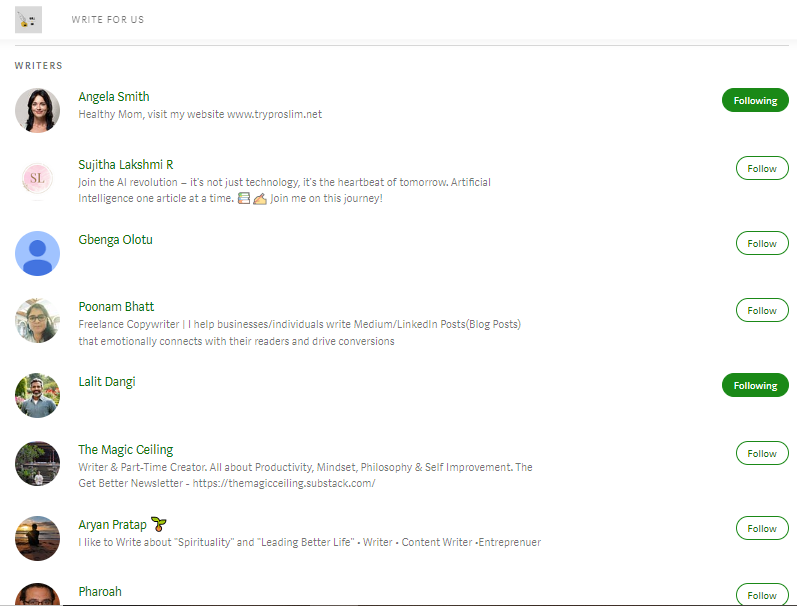The screenshot depicts a webpage from a writing platform with a "Write For Us" section prominently displayed in the top left corner, just above a light gray navigation bar. Below this, there's a section labeled "Writers" featuring a list of contributors along with their brief profiles, avatars, and follow buttons.

1. **Angela Smith**: Her profile includes a picture of a woman. The description reads "Healthy Mom," followed by a link to her website: [www.tryproslim.net](http://www.tryproslim.net). The follow button next to her profile indicates she is already followed and is colored in a dark green.

2. **Tsuhita Mashimi-R**: This profile features an initial-based logo as the avatar. The description is vibrant, stating: "Join the AI revolution. It's not just technology; it's the heartbeat of tomorrow, artificial intelligence, one article at a time." It is interspersed with book and writing emojis. It ends with "Join me on this journey," inviting users to follow her.

3. **Benga Ulutu**: Displaying a default profile picture, this user's profile has no additional description and features a follow button.

4. **Poonam Bot**: Her profile entails a picture of a lady and reads: "Freelance copywriter. I help businesses/individuals write Medium/LinkedIn posts, blog posts that emotionally connect with their readers and drive conversations." A follow button is available next to her description.

5. **Lilit Dongi**: This profile features a picture of a man but lacks a description. The button next to it indicates this user is being followed.

6. **The Magic Ceiling**: The profile includes a photo with no specific person shown. The description reads: "Writer and part-time creator. All about productivity, mindset, philosophy, and self-improvement. The write better newsletter," followed by a link to their Substack page titled "The Magical Ceiling." There is an option to follow as well.

7. **Aryan Pratap**: The profile features a photo of a person against a sunset background and includes a plant emoji. The description reads: "I like to write about spirituality and leading a better life. Writer, content creator, entrepreneur." A follow button is available next to it.

8. **Farrow**: Identified as "partially sane" and providing minimal information, this profile also comes with a follow button.

Each writer's profile is accompanied by easy-to-click follow or following buttons, ensuring users can connect with their favorite authors conveniently.